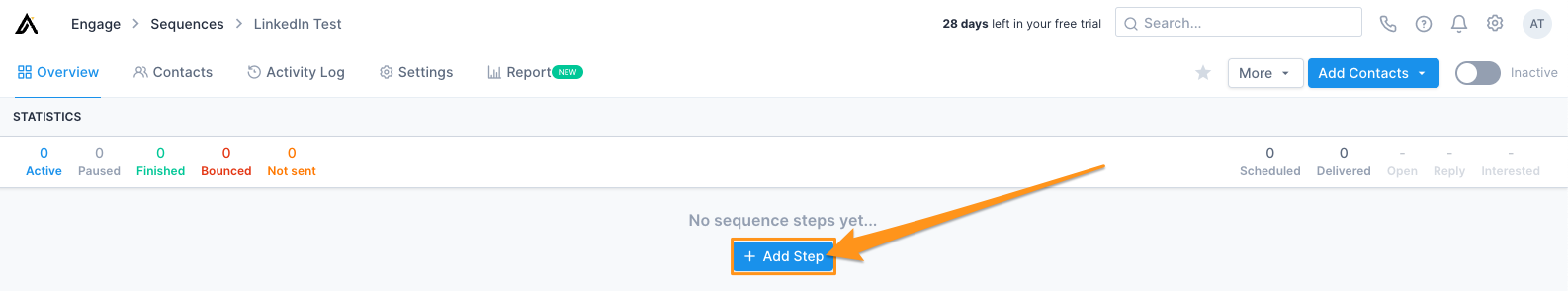The screen displays an interface for a statistics program within an application. At the very top, there's a navigation path reading "Engage > Sequences > Linkedin Test." To the far right, a notification informs the user that they have "28 days remaining in your free trial," positioned next to an empty search bar. Adjacent to the search bar are a series of icons: a phone, a question mark, an alarm bell, and a settings gear, along with a gray circle bearing the initials "AT."

On the second line, the "Overview" menu option is highlighted, and directly below, the word "Statistics" is prominently displayed. The statistics section displays five categories, each marked with a '0’: "0 Active," "0 Paused," "0 Finished," "0 Bounced," and "0 Not Sent."

The main portion of the screen poignantly features the text "No Sequence Steps Yet..." accompanied by a blue button with a plus sign, labeled "Add Step." The button is accented by an orange arrow, serving to highlight it and draw the user's attention.